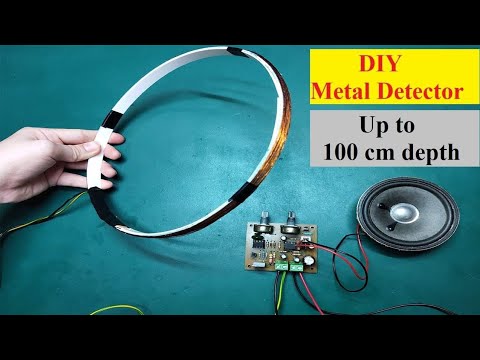The image is a color photograph framed by black borders at the top and bottom. It features a dark aqua background. On the left side, a hand is holding a large, round piece of metal, which appears to be a hoop with various colors such as silver, black, and gold, and possibly wrapped with electrical tape. Copper wires are attached to the outer edge of the hoop. To the right of this, there is a yellow rectangle with red text stating "DIY Metal Detector." Beneath this, in a gray box with black letters, it states "Up to 100cm Depth." Below these text boxes, the photograph showcases a speaker lying on the aqua background. The speaker has black and red wires connected to a circuit board, which also has additional black, red, and green wires trailing from it. The overall impression is that this image could be part of instructional content for assembling a homemade metal detector.